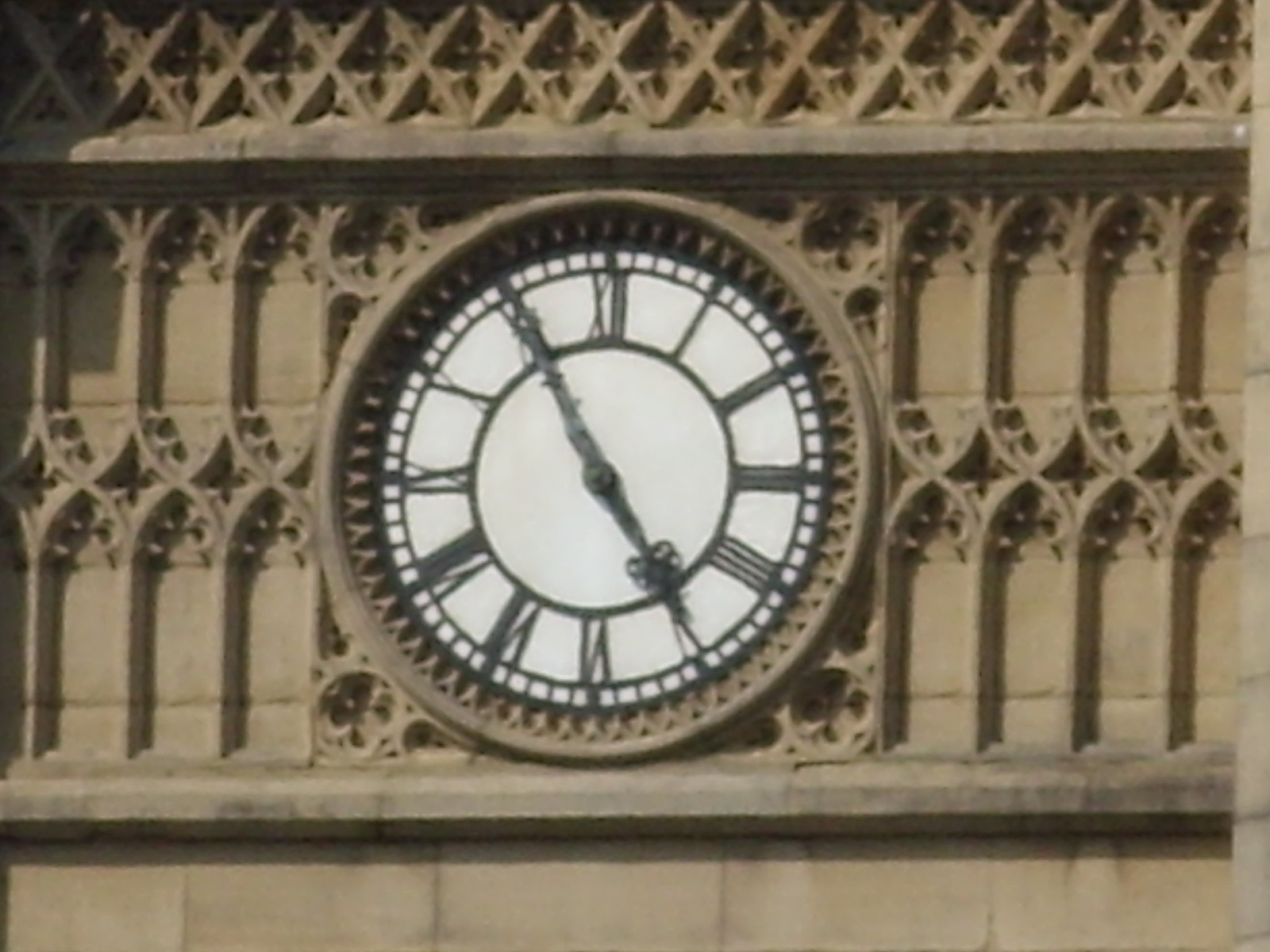This photograph captures an intricate wall clock mounted on the side of a tall, aged building, likely constructed of grayish-brown stone. The clock face, featuring bold black Roman numerals and encircled by two concentric black rings, is bordered by a white rim with black trim. The ornate black hands, resembling cast iron, indicate the time as 4:55. Surrounding the clock is an elaborately decorated facade with vertical repeating geometric patterns, characteristic of old architecture, suggesting the building may be over a hundred years old. Above the clock, a stone ledge runs along the top of the image, adorned with approximately twenty repeating cross-sword motifs, adding to the historic and decorative nature of the structure. The photograph, seemingly taken with a telephoto lens, reveals fine details but is somewhat fuzzy, indicating it was shot from a considerable distance.